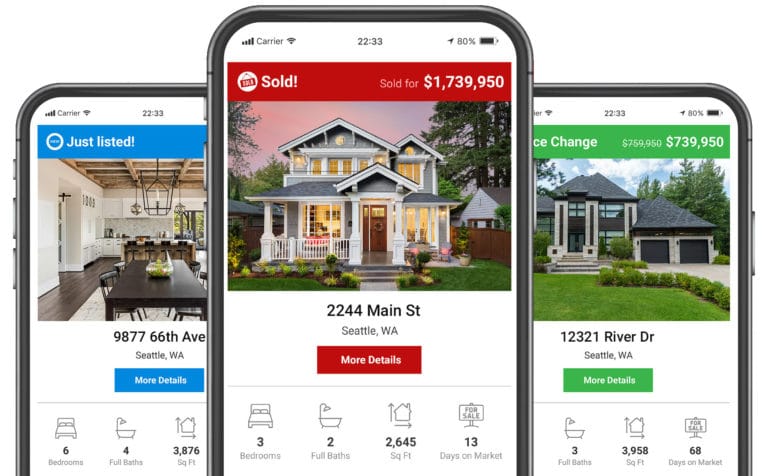This image is a composite screenshot of three different phone screens, each displaying property information related to houses in Seattle, Washington. 

The first screenshot, situated on the left, features a listing from a real estate app with a blue top banner stating "Just Listed." It showcases an interior photo of the dining room of a house located at 9877 66th Avenue. The house boasts six bedrooms, four full bathrooms, and a generous living space of 3,876 square feet. The image captures a modern dining room with a black table, and the timestamp on the screen indicates 22:33, or 10:33 PM.

The middle screenshot also shows a timestamp of 22:33. This one has a red top banner labeled "Sold." The property in question sold for $1,739,950. The image in this screenshot displays an external view of a three-level house that appears spacious and well-maintained.

The third screenshot on the right appears to be cut off, but it features a property with a recorded "Price Change." The banner is partially visible, and the property’s price has been adjusted from $759,000 to $739,000.